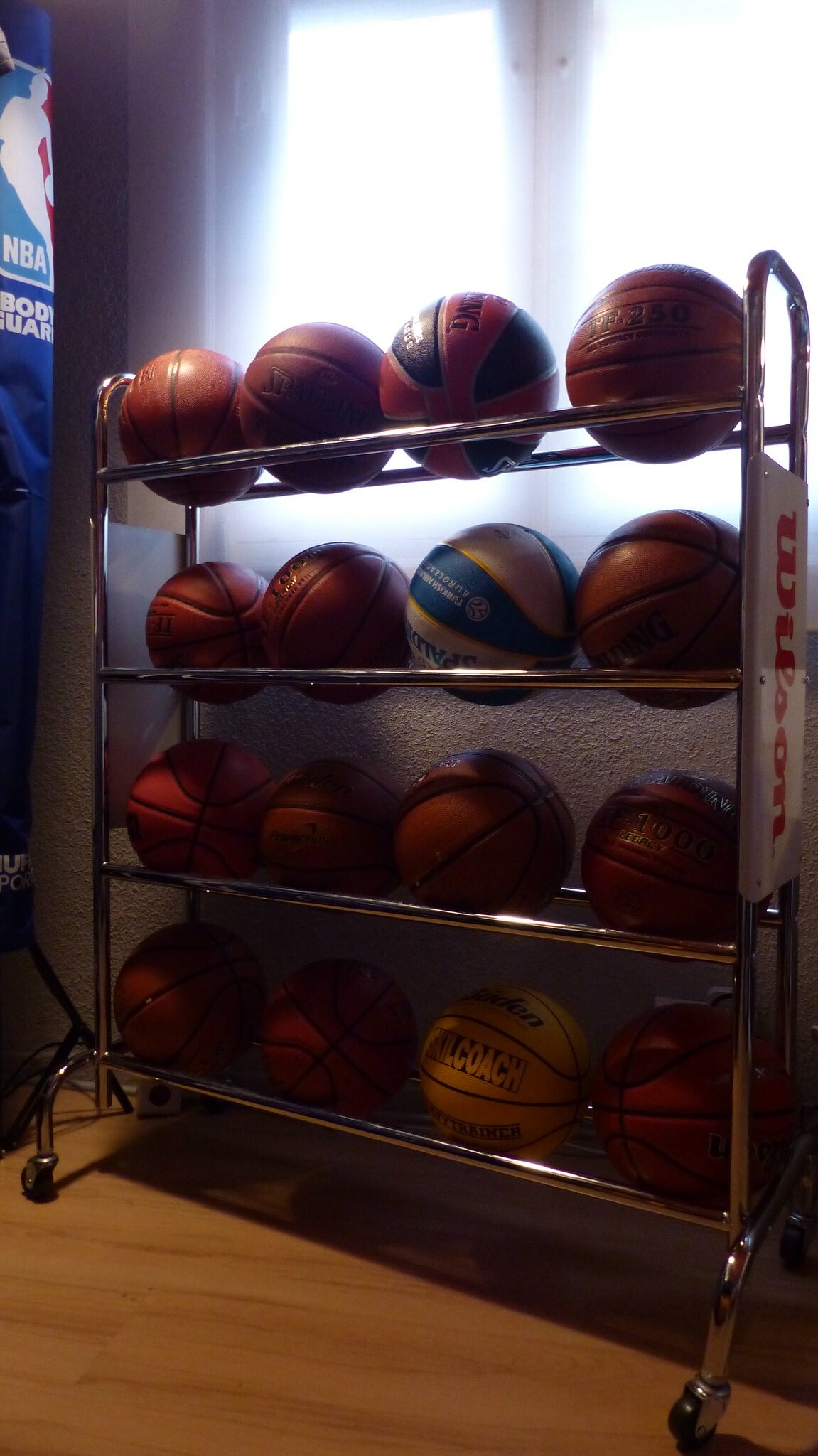In this detailed image, a metal rack made of silver-colored tubes and equipped with black wheels holds an organized assortment of sixteen basketballs. The rack features four shelves, each containing four basketballs, aligned in neat rows. Most of the basketballs are the traditional orange color, while some have distinct yellow, blue, white, and red stripes. The sturdy rack prominently displays a sideways "Wilson" logo, indicating the brand of the equipment. This setup is situated on a light brown wooden floor, against what appears to be a white brick or concrete wall, illuminated by two columns of light casting down directly on the balls. In the background, partially out of view, a blue and white sign with the "NBA" logo can be seen, hinting at the professional quality of the facility, which resembles an indoor gymnasium. The photographer captured this organized display from the front, emphasizing the array of basketballs gleaming under the gym lights.